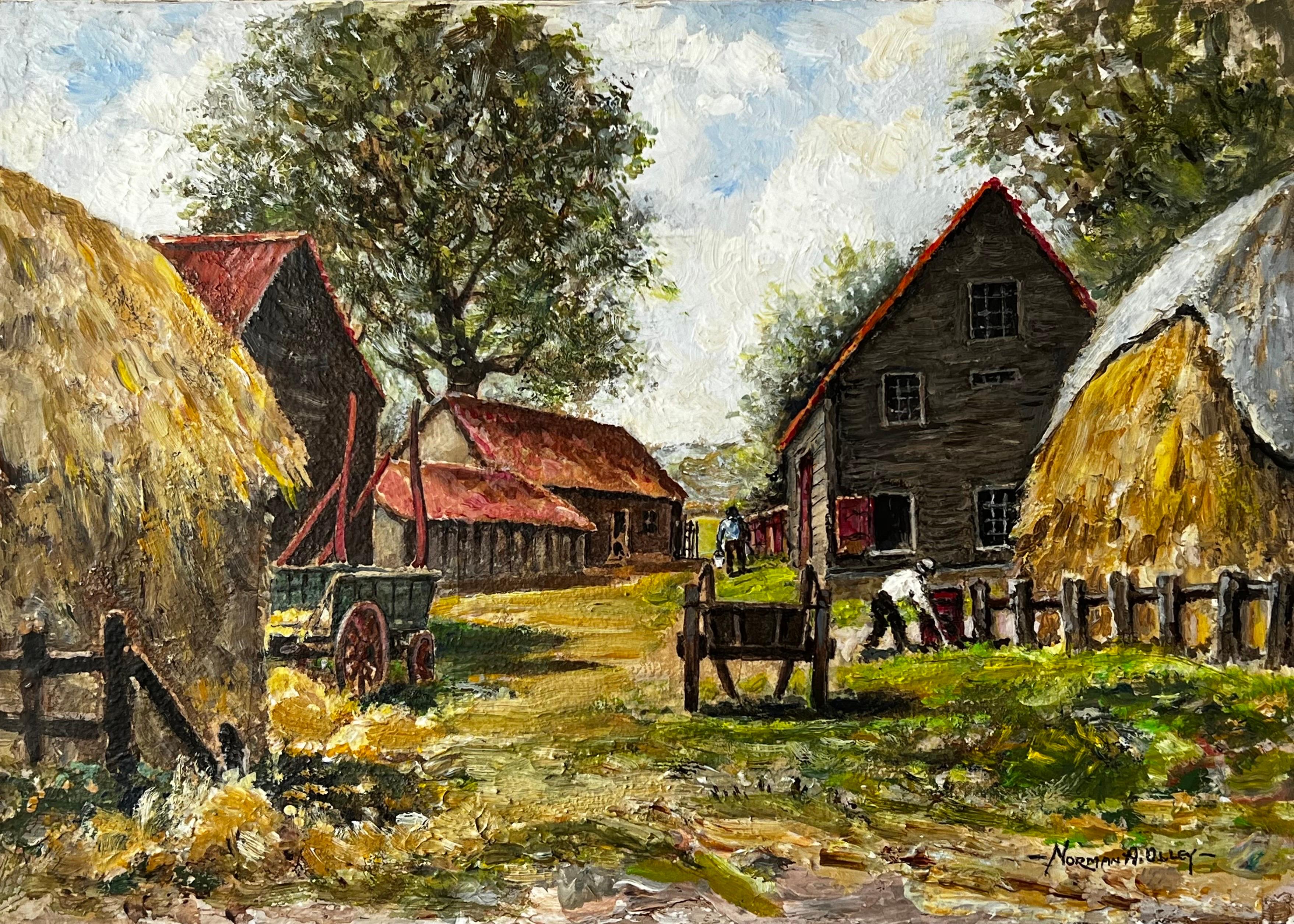This horizontally wide painting, potentially an oil piece with textured spots, is signed by Norman A. Ollie in the bottom right corner. It captures a pastoral scene, suggesting an earlier era with large brown buildings featuring red roofs. In the background, there are two prominent, tall trees with another smaller one barely visible over the roof of one house. Two significant haystack structures lie on either side of the scene. The one on the left, partially obscuring a wheelbarrow with red wheels and a blue base, is bordered by a brown wooden fence. The right-side haystack also sits behind a similar wooden fence.

To the far left, near a large haystack structure, a man wearing a white shirt and black pants is seen tending to the haystack. This rustic tableau is further detailed with various agricultural elements like farm tools and vehicles. The ground is a mosaic of yellow, brown, and green shades, indicative of cultivated land.

The sky in the background is light blue, mostly covered in white clouds, maintaining a clear, serene atmosphere. The image vividly conveys a time when people worked the land, underscored by the absence of modern roads and the presence of numerous farm buildings, structures, and large overshadowing trees.